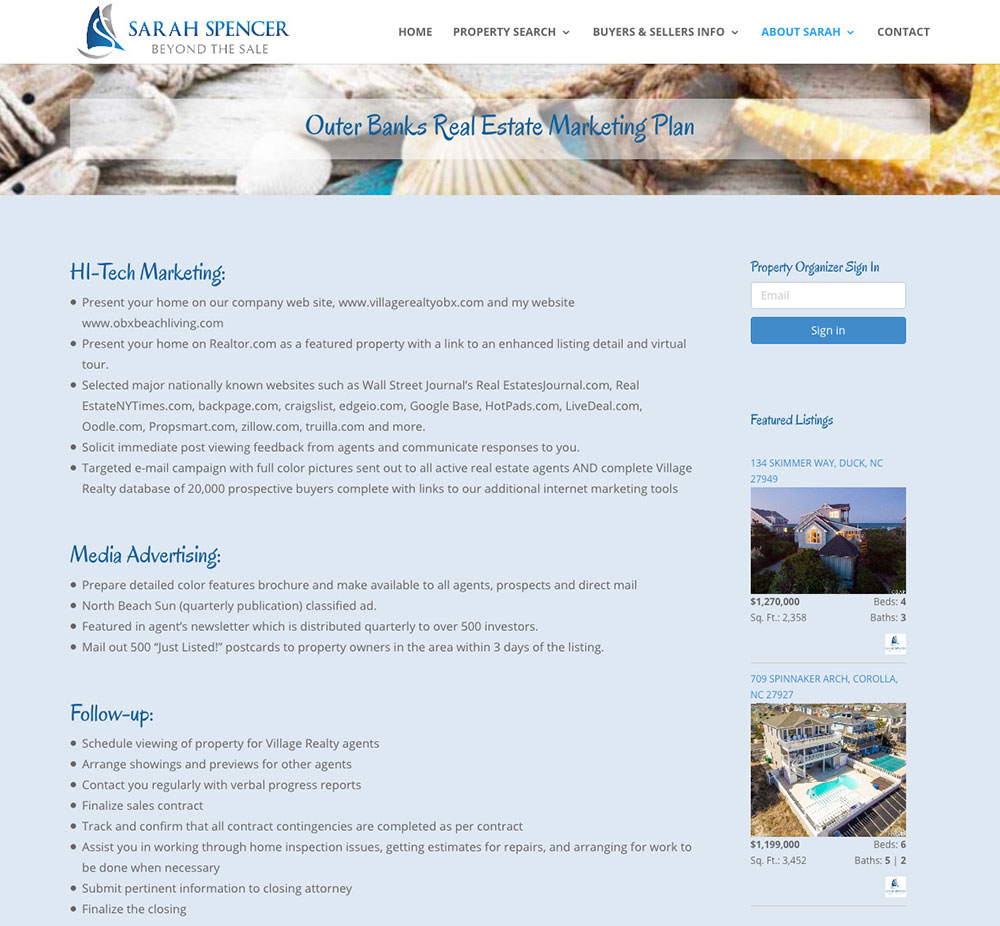This is an image from the website "Sarah Spencer Beyond the Sail," which serves as an online platform for Sarah Spencer, a real estate professional specializing in the Outer Banks area. The site's design prominently features Sarah Spencer, who is depicted wearing blue clothing. The image showcases an elegant aesthetic that includes two sail-like shapes in blue and gray, accompanied by a swirl underneath, possibly symbolizing a sailboat theme.

The website's primary sections are categorized under various research topics, including: Home, Property Search, Buyer's and Seller's Info, About Sarah, and Contact—each title highlighted in blue. This organization suggests that Sarah is a seasoned realtor with a focus on comprehensive real estate services.

Central to the image is the "Outer Banks Real Estate Marketing Plan," set against a visually pleasing backdrop featuring large seashells, a starfish, and a piece of driftwood, all evoking a coastal theme. This marketing plan is encapsulated in a clear white box with elegant blue lettering. Below this title, a greyish-blue box introduces the "High-Tech Marketing" section with five black bullet points detailing various aspects of the marketing strategy. For example, it mentions presenting your home on both the company's and Sarah's individual websites.

Additional sections of the image include "Media Advertising" and "Follow-Up," each accompanied by bullet points and detailed explanations. There is also a "Property Organizer" section, where users can input their email address to sign in, encouraging engagement.

Towards the bottom, a blue bar highlights "Featured Listings," showcasing two available properties with beautiful accompanying photographs. This layout not only provides a comprehensive overview of Sarah Spencer's real estate services but also emphasizes a high level of professionalism and attention to detail in marketing homes.